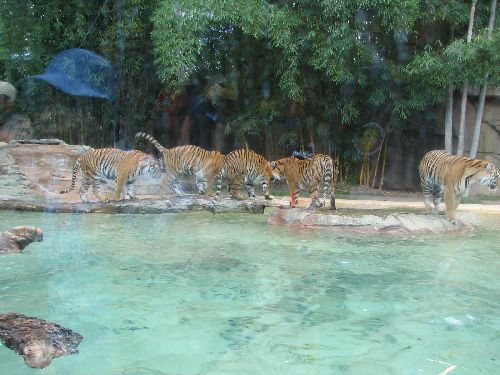The image, captured at a zoo, depicts a group of five tigers in their enclosure, with the scene viewed through protective glass, evidenced by slight reflections. The background features a dense curtain of tall, dark green trees, providing a naturalistic setting for the tigers. The enclosure contains an expansive body of calm, light turquoise water, which occupies the lower half of the frame and stretches from one side of the image to the other.

The tigers, characterized by their distinguished orange and black fur, are positioned on light yellow and gray-brown rocks that border the water. The animals are captured at various angles; one tiger on the right stands near the water's edge, facing slightly towards the viewer, while the other four are grouped together, looking sideways and appearing to be mid-stride. The scene’s clarity is somewhat compromised as the tigers appear slightly blurry, likely due to the glass’ protective nature. The glass also reveals a faint reflection in the top left corner of a person wearing a blue hat.

Further detail includes the rugged, rocky terrain that transitions into a mix of light yellow and light brown stones both inside and around the water. Additionally, the right side of the enclosure includes a visible structure, possibly a shelter for the tigers. The stones within the water appear hard and gray, contrasting with the water’s pale aqua hue. Overall, the composition balances natural elements and the zoo’s constructed environment, highlighting the tigers both in the context of their habitat and the viewing experience facilitated by the enclosure's design.